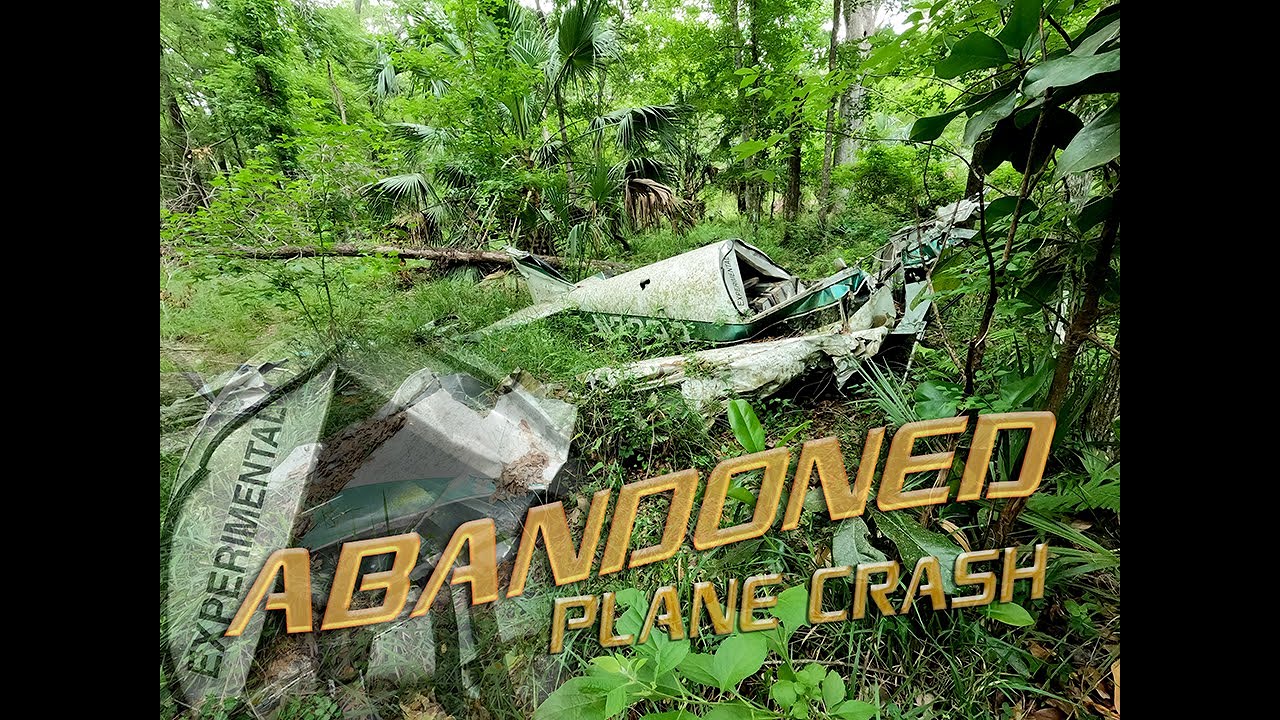This detailed photograph, set in a landscape orientation, features a dramatic and eerie scene of an abandoned plane crash nestled deep within a lush, tropical jungle. The image measures approximately 6 inches wide and 3 inches high, bordered by half-inch black strips on the left and right sides. In the photograph's center, the shattered fuselage of a white airplane with a prominent green horizontal stripe is visibly crumpled on the jungle floor. The damaged aircraft is marked with the word "experimental," prominently displayed on the broken-open part of the fuselage, as highlighted by an inset overlay in the lower left-hand corner. The tail of the airplane is clearly discernable, showing both the vertical and horizontal fins amidst the dense foliage of palm trees and tropical plants. Adding to the somber mood, the phrase "abandoned plane crash" is inscribed in gold, wavy text across the bottom of the photograph.